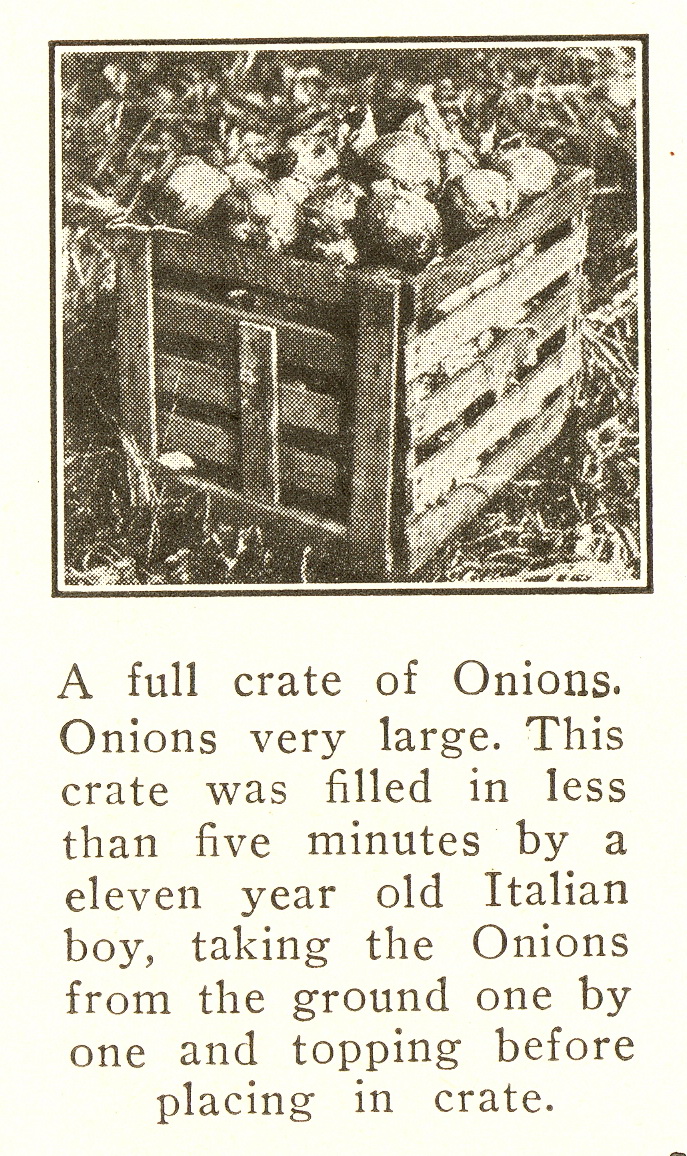The image appears to be an aged newspaper or magazine clipping with a creamy background. At the top of the clipping is a grainy black and white photo, bordered first by black and then by white. This photo captures a square, wooden crate filled to the brim with large onions, set against a grassy backdrop. The text underneath the image, in light black writing, reads: "A full crate of onions. Onions very large. This crate was filled in less than five minutes by an 11-year-old Italian boy, taking the onions from the ground one by one and topping before placing in the crate."